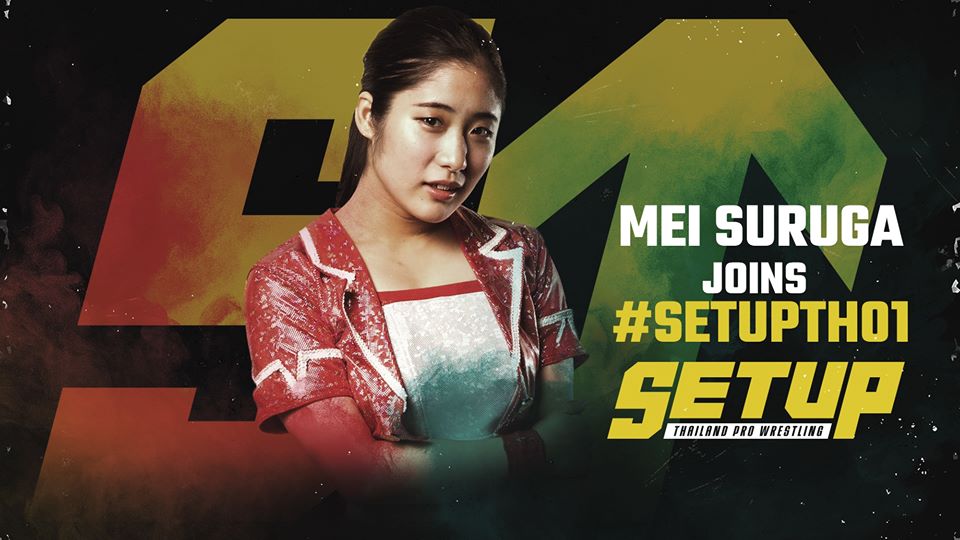A vibrant promotional image features an Asian woman with black hair pulled back, adorned in a sparkly red jacket with white accents on the sleeves and collar, and a white shirt that sports a red horizontal stripe. She stands confidently, facing the viewer against a night sky-like black background scattered with white stars. Central to the image is a bold logo depicting an "S" and an upward-pointing arrow in a palette of red, green, orange, and yellow. To her right, text in white announces "May Suruga joins" above a yellow hashtag "set up th01," followed by the phrase "set up" and "Thailand Pro Wrestling" underneath. The entire composition beams with a multitude of colors, including tan, brown, black, and pink, enhancing its dynamic appeal.